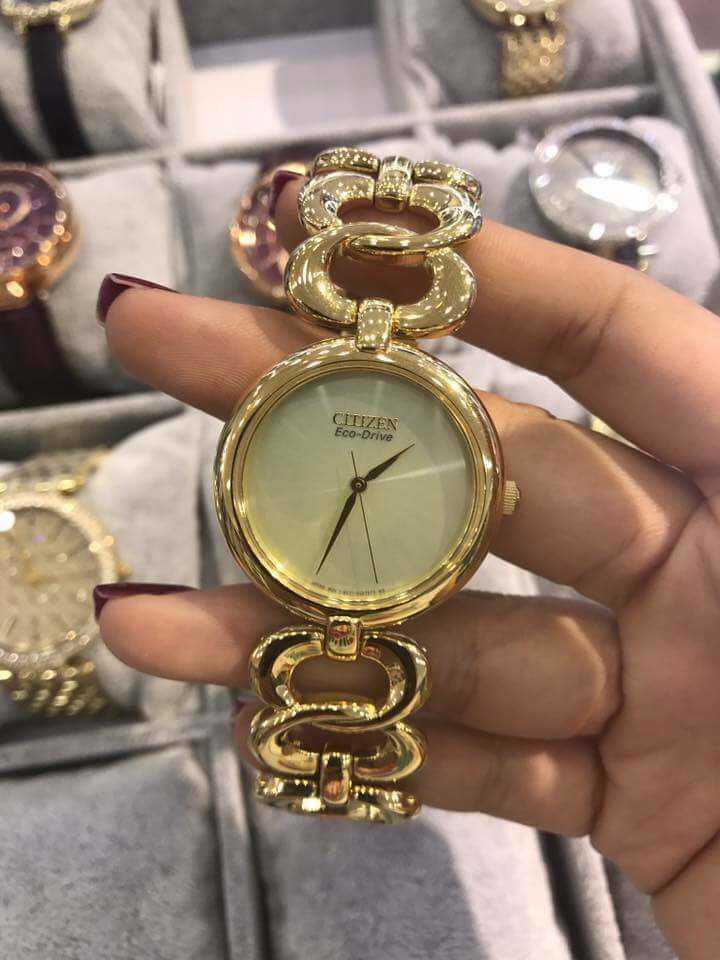In this color photograph, we see a close-up of a woman's hand with maroon fingernail polish, holding a stunning, elegant gold Citizen Eco-Drive wristwatch. The hand, visible from the lower fingers and palm, prominently displays the watch, focusing the viewer's attention. The watch features a round, tan dial with gold and black accents, including gold hour, minute, and second hands. It is approximately 1:35 on the watch face. The Citizen logo is proudly displayed at the top of the dial. Encircling the wrist are delicate yet wide interlocking gold circles, forming the band. A gold knob protrudes from the right side of the case, used for adjusting the time. In the blurred background, there are other wristwatches displayed on gray, padded deck displays, suggesting a store setting. A variety of watches with different face colors and gold details can be seen, adding depth to the image but keeping the gold Citizen wristwatch as the focal point.